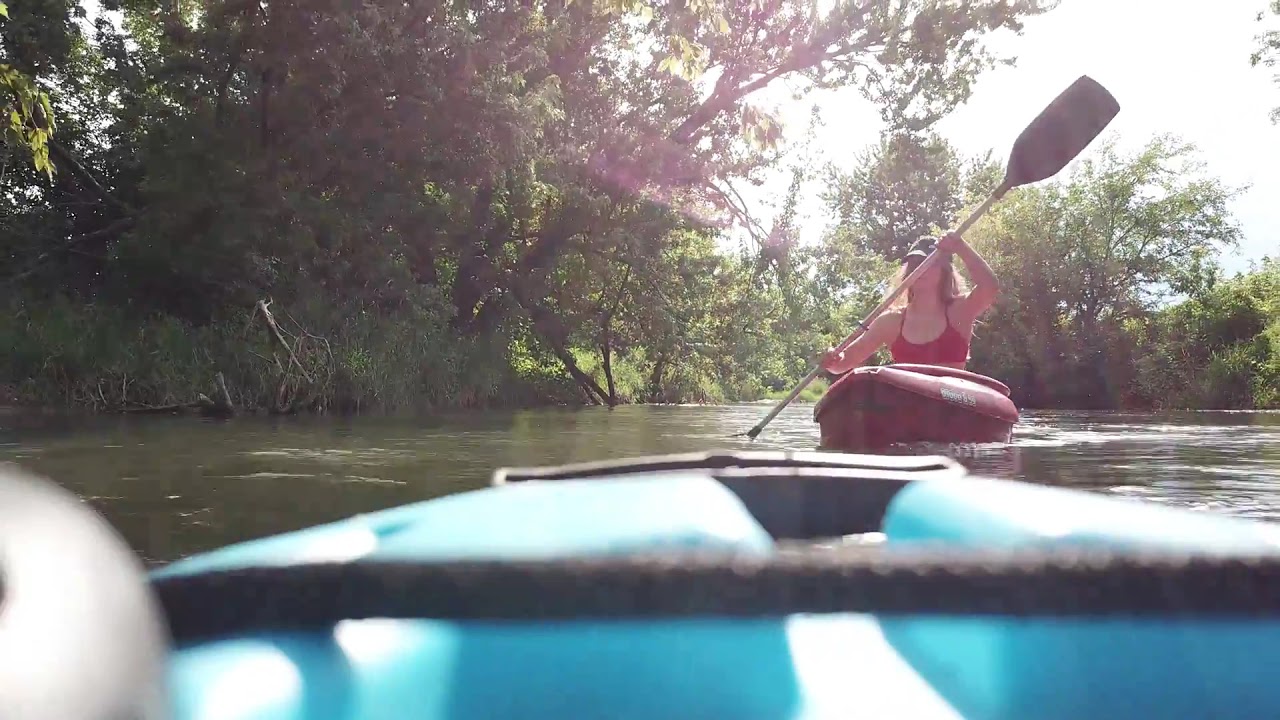This image captures a serene water activity scene from the perspective of someone sitting in a blue kayak. In the foreground, the tip of the blue kayak is visible, hinting at a mix of calm water and light ripples caused by paddling. Directly ahead, a woman in a small red kayak commands attention. She is actively paddling towards the camera with a large oar. The woman is wearing a red swimsuit and a brown hat, her focus clearly on navigating through the water. The water appears fairly calm, reflecting a partly cloudy sky, though it has a somewhat muddy hue synonymous with a creek. Surrounding this tranquil scene is lush greenery, including trees and shrubs, which create a natural backdrop. The greenery is so dense and shapely that some of the shrubbery mimics the iconic silhouette of the Eiffel Tower. The overall color palette of the image is dominated by blues, reds, and earthy greens, providing a vibrant yet serene visual experience.